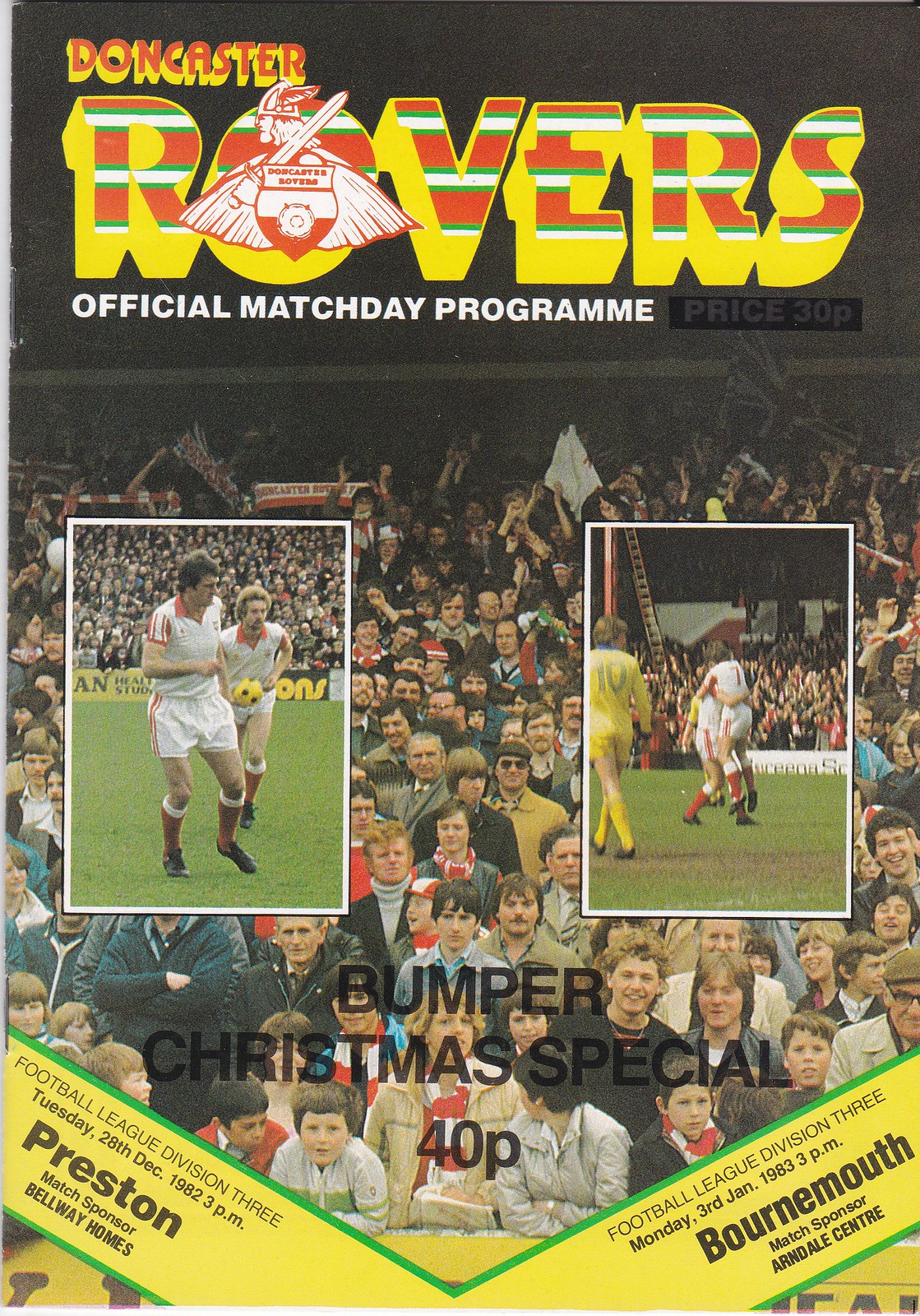This image is a detailed sports program cover for the Doncaster Rovers. At the top, "Doncaster Rovers" is prominently displayed in bold yellow and orange type. An official match day program header sits below, featuring a soldier-like mascot perched on the 'O' of "Rovers." The program is the bumper Christmas special, priced at 40p. 

The central background showcases a large photo of spectators in a stadium, creating an immersive atmosphere. Overlaid on this are two action shots: one on the left, depicting two soccer players in white uniforms with red stripes and red socks, in the midst of a play; and one on the right, showing two players in white and red uniforms, one of whom is number 7, celebrating together. In this scene, there is also a player from the opposing team in a yellow jersey, marked with the number 10.

A yellow V-shaped banner at the bottom provides essential match details. On the left side, it reads:

- "Football League Division III
- Tuesday, 28th December 1982, 3 p.m.
- Preston
- Match Sponsor: Belway Homes."

On the right side, it states:

- "Football League Division III
- Monday, 3rd January 1983, 3 p.m.
- Bournemouth
- Match Sponsor: Arndale Centre."

The cover is vibrant with colors including red, white, green, blue, black, yellow, and orange, painting a vivid depiction of the spirited soccer event.